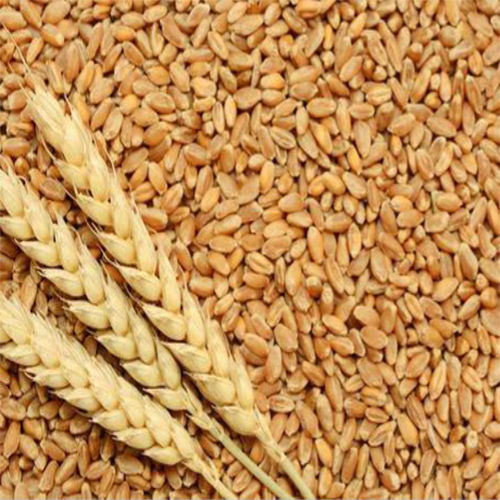The image captures a square close-up of a massive pile of wheat kernels, covering the entire frame with their light to medium brown hues. The kernels create a textured background, reminiscent of grains just harvested and unprocessed. Staged carefully, three lighter tan wheat plants are prominently placed in the bottom left corner, angled upward to the left. These plants, with their slender stalks and clusters of wheat kernels, contrast with the darker pile beneath them. The photograph, which contains no text, showcases the varied shades of brown and tan, highlighting the natural tones and intricate details of both the pile of kernels and the wheat plants.